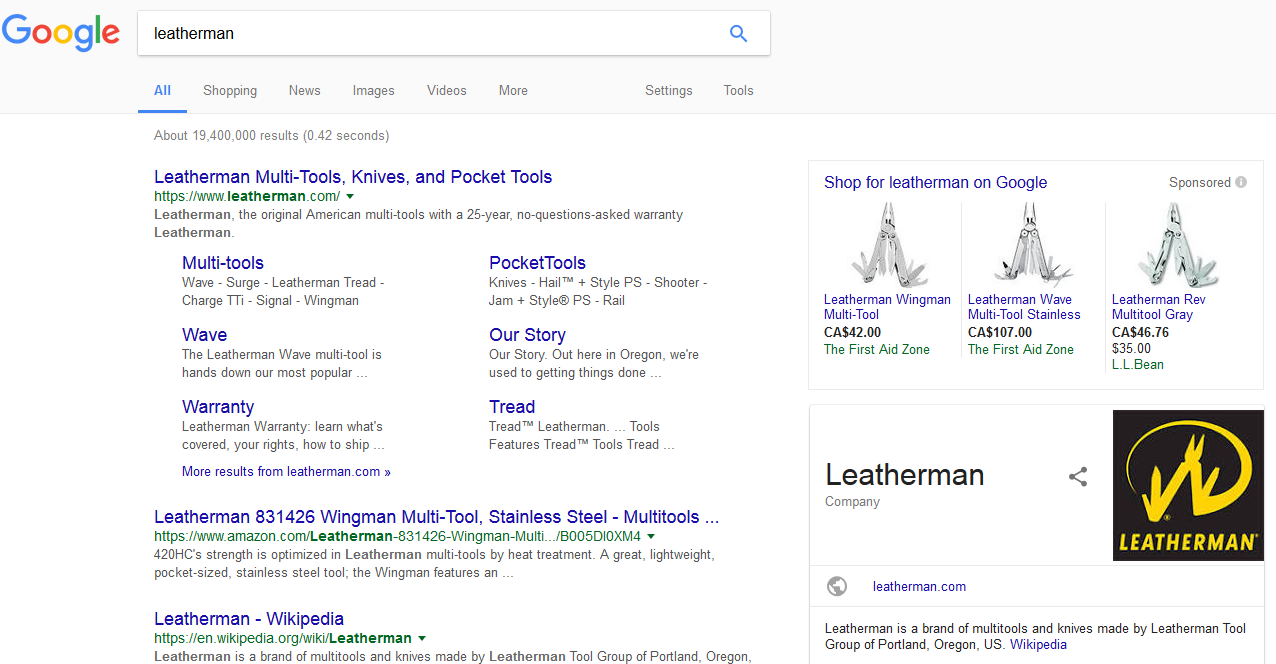This image displays a Google search results page. Featured prominently in the upper left corner are Google's iconic colors: blue, red, yellow, and green. The search query entered is "Leatherman," visible in the primary search field.

Directly underneath the search bar, several navigation options are listed: All, Shopping, News, Images, Videos, More, Settings, and Tools. Notably, there is no "Music" tab mentioned. 

The search engine indicates approximately 19,400,000 results were found in 0.42 seconds. The first result listed is for Leatherman multi-tool knives and pocket tools from leatherman.com. It highlights Leatherman as the original American multi-tool brand, boasting a 25-year no-questions-asked warranty. Several keywords are emphasized: multi-tools, warranty, pocket tools, and our story.

Further results include specific product listings, such as the Leatherman 831426 Wingman multi-tool in stainless steel available on Amazon, as well as a Wikipedia entry that provides an overview of the Leatherman brand, which is manufactured by the Leatherman Tool Group in Portland, Oregon.

On the right side of the page, there is a row of three images showcasing various Leatherman products. Most of these images are associated with listings from first aid sites and depict different Leatherman multi-tools.